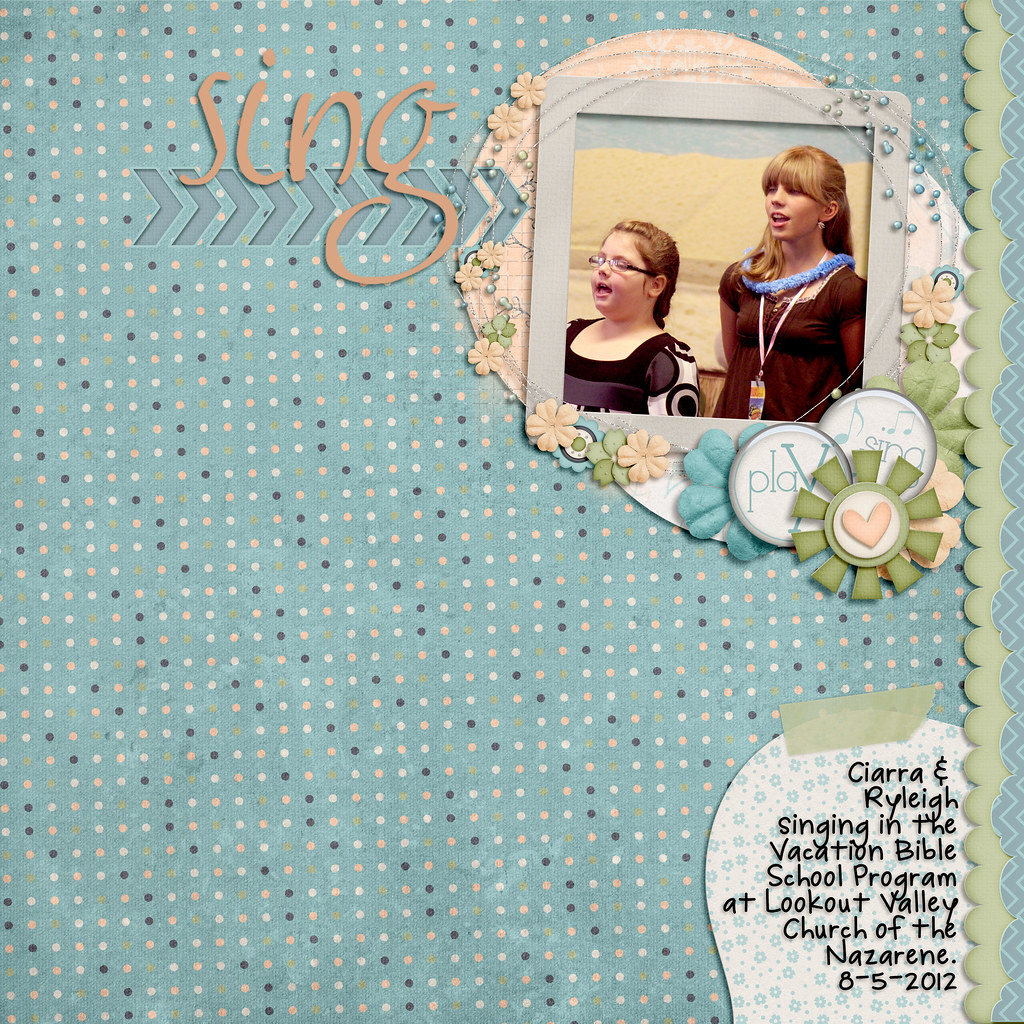The image is a page in a scrapbook journal with a light green background adorned with peach and darker green polka dots. At the top, there's the word "sing" accompanied by a decorative border framing a photograph of two girls. The girl on the right has bangs and her hair pulled back, wearing a maroon dress with a lanyard around her neck, and appears to be singing. The other girl is shorter, wears glasses and a black and white dress, and also looks like she is singing. Below the photo are decorations, including flowers and a circle that says "play and sing." In the bottom right corner, black text reads, "Sierra and Riley singing in the Vacation Bible School program at Lookout Valley Church of the Nazarene, 8-5-2012."